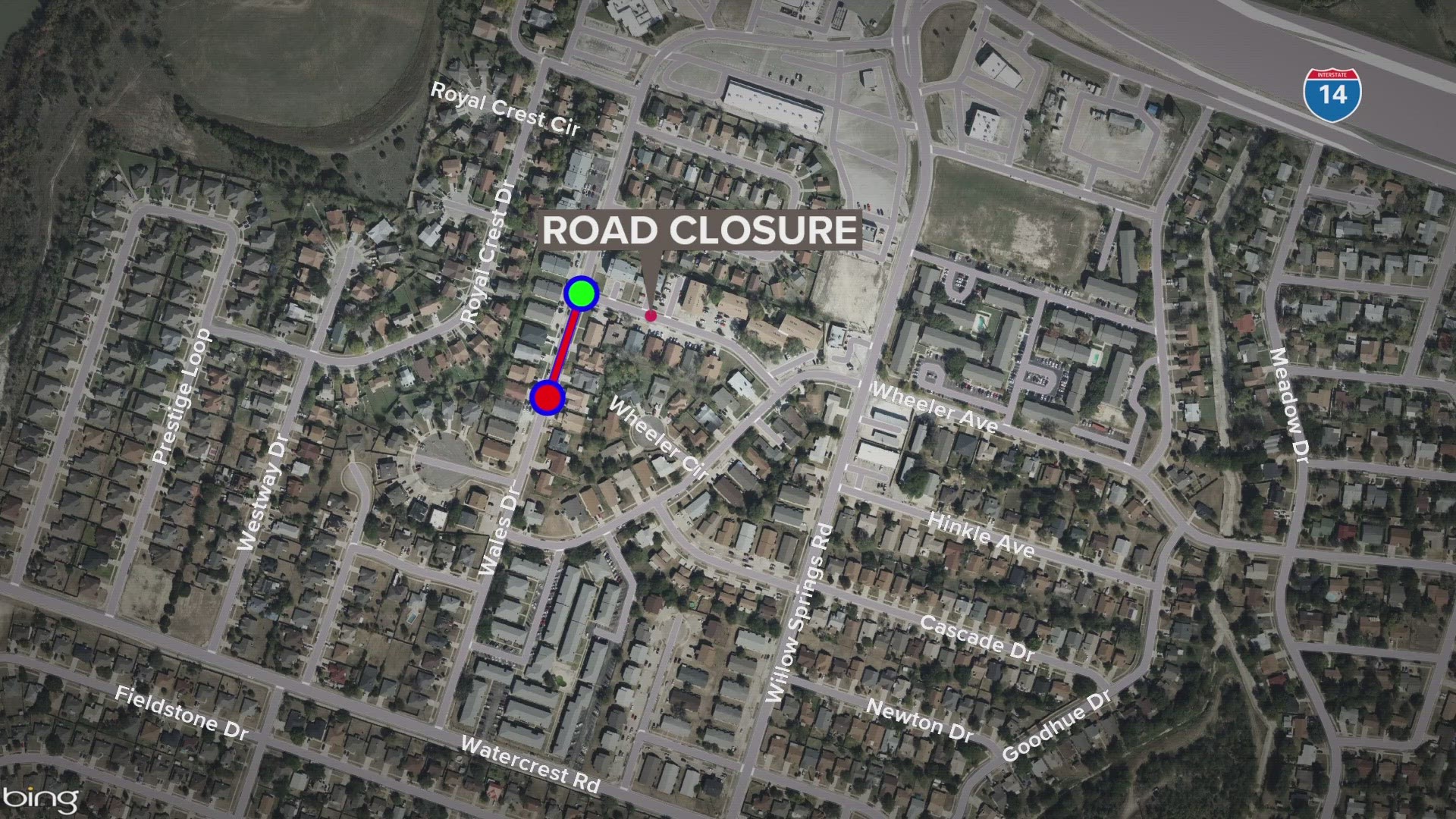This image depicts a detailed aerial view of a housing district, captured from what appears to be Bing Maps, as indicated by the Bing logo in the bottom left corner. The entire image presents a grayscale map displaying various houses, streets, and road names, generating the feel of a satellite or aerial photograph. Key road names visible include Prestige Loop, Fieldstone Drive, Westway Drive, Wales Drive, Watercrest Road, Willow Springs Road, Newton Drive, Goodhue Drive, Wheeler Avenue, Meadow Drive, and Royal Crest Circle, written in white font. 

A notable feature in the middle of the image is a gray marker indicating a "Road Closure," highlighted by the text 'road closure' in white with a gray border around it. Additionally, a green dot outlined in blue is connected via a red line to a red dot also outlined in blue, signifying another area of interest. Nearby, another red dot can be observed. On the top right corner, a logo resembling a shirt displays the text "Interstate 14" with 'Interstate' written in red and '14' in blue.

The image is rich with small details, such as the positions of houses, roads, and the specific markers indicating a road closure, adding depth to the depiction of this urban or suburban landscape.